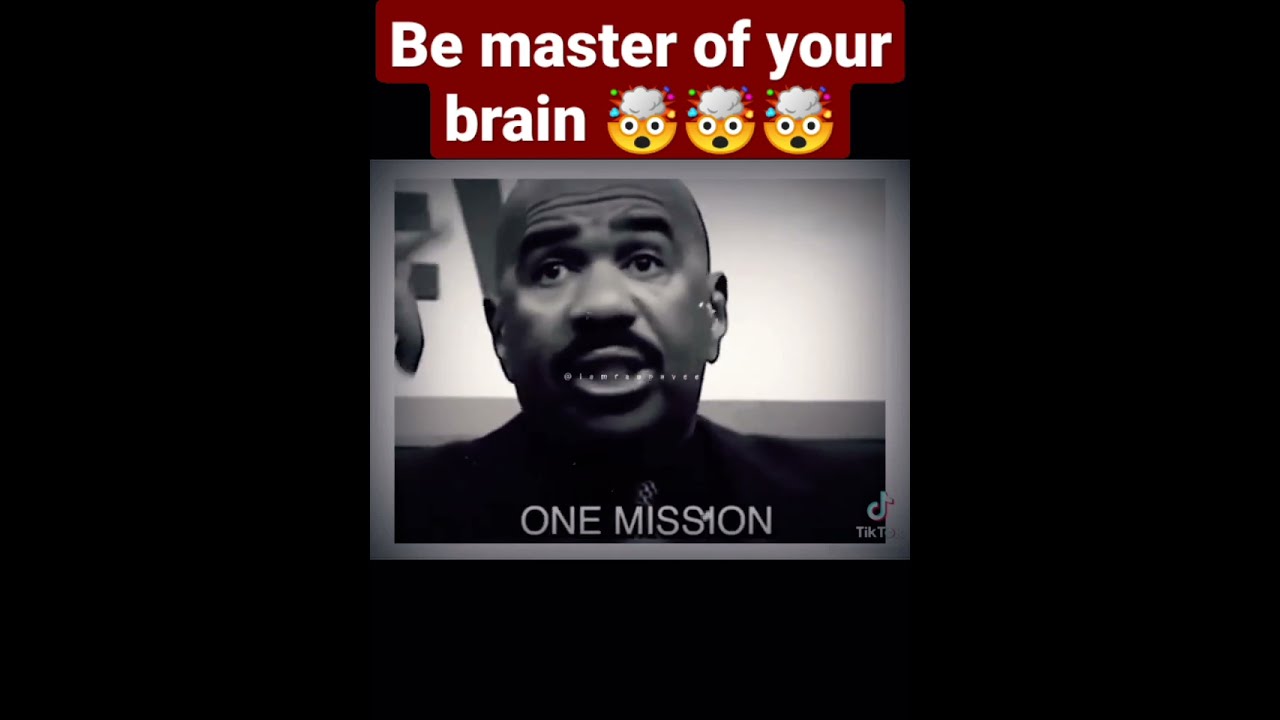The image is a black and white photograph set against a black background. At the top of the image, there's a maroon-colored strip with bold white text that reads "Be Master of Your Brain," accompanied by three mind-blown emojis featuring wide eyes, open mouths, and clouds at the top of their heads. Below this text, there's a black and white picture of the comedian Steve Harvey. He has a bald head, mustache, bushy eyebrows, and appears to be wearing a dark suit jacket and necktie. His mouth is open as he looks straight ahead. The picture of Steve Harvey is bordered by a gray frame, and in the bottom right-hand corner sits the TikTok symbol. Below the image is a caption in white text that reads, "One Mission."